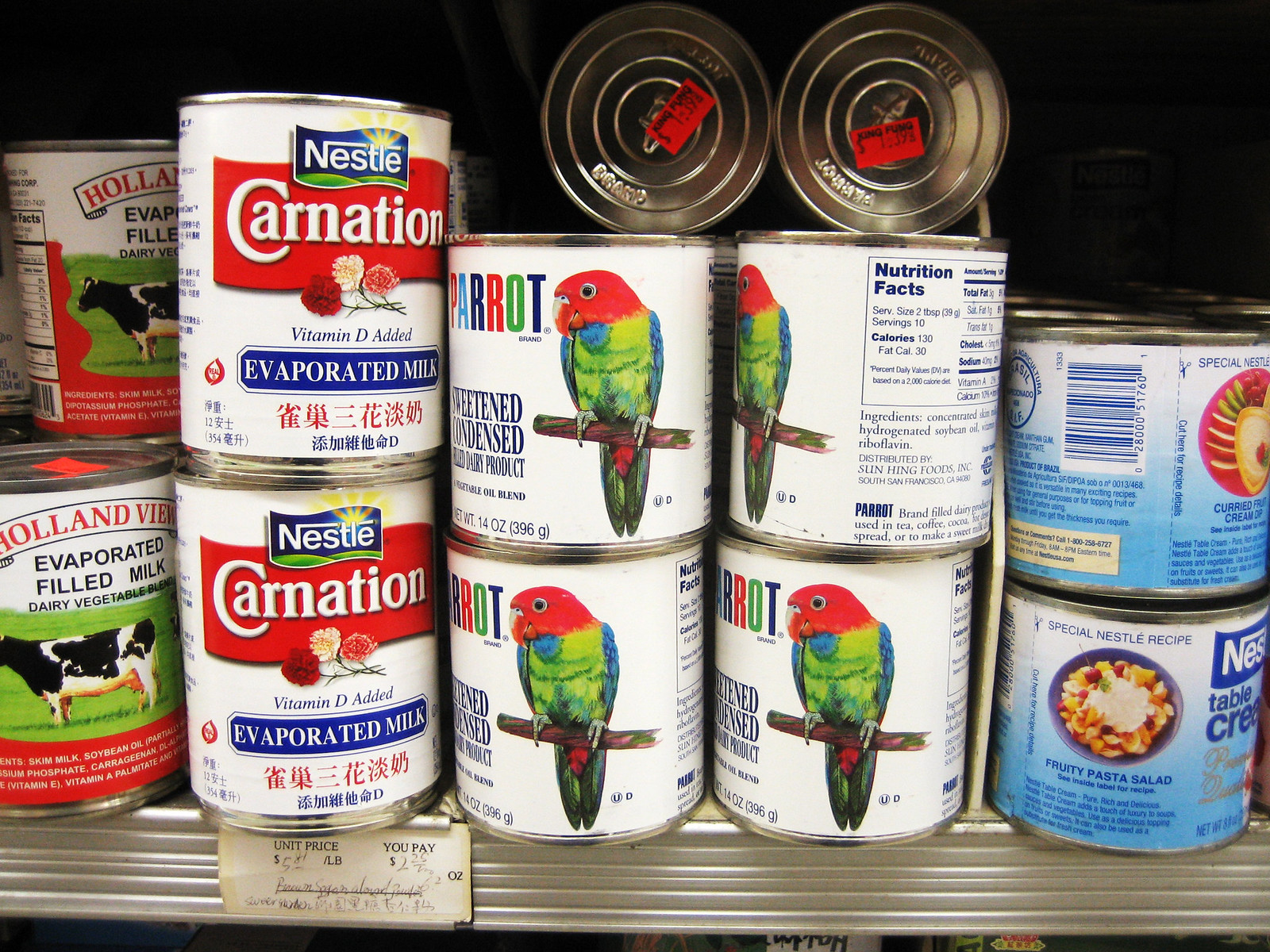The image depicts a supermarket shelf lined with several types of evaporated and sweetened condensed milk cans, arranged in neat vertical stacks. The scene includes:

- **Left Section**: Two cans of "Holland View Evaporated Filled Milk," each featuring a black and white dairy cow positioned in a green field. The label includes the product name in white text against a red background.
  
- **Middle Section**: Two cans of "Nestle Carnation Evaporated Milk" with added Vitamin D, identifiable by their predominantly white labels with a red banner where the word 'Carnation' is written in white. The labels also feature red, white, and pink carnation flowers.
  
- **Next Section**: Four cans of "Parrot Sweetened Condensed Milk." Each can showcases a vibrantly colored parrot with a red head, an orangey-green stomach, and blue wings, perched on a branch. The label is prominently multi-colored.
  
- **Right Section**: Two smaller cans of "Nestle Table Cream." The cans have blue labels, with the bottom can displaying an image of a pasta salad and the top can partially showing the barcode.

The metal cans rest on a metal shelf, highlighting the interior setting of a grocery or convenience store.